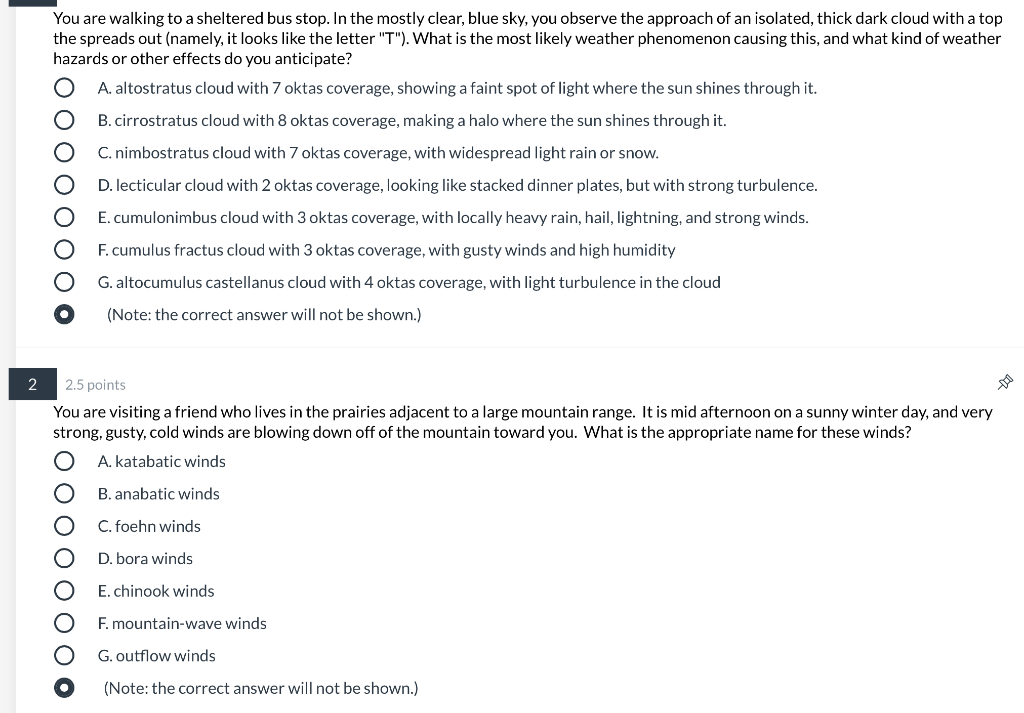The image depicts a clean and simplistic web page with a completely white background, adorned with a significant amount of black text. At the very top, there is a narrative scenario: "You are walking to a shattered bus stop under a pristine blue sky. During your walk, you notice the approach of an isolated thick dark cloud that spreads out at the top, resembling the shape of the letter 'T'. What is the most likely weather phenomenon causing this, and what kind of weather hazards or other effects do you anticipate?"

Following this narrative, there are multiple-choice options labeled from A to G, each describing different weather phenomena. The first option, A, reads: "Altostratus clouds with seven-eighths coverage, showing a faint spot of light where the sun shines through." Below each option are white dots that can be clicked. 

A note beneath this section indicates: "Note: The correct answer will not be shown."

Further down, the web page contains another numbered scenario, marked as "2" with a value of "2.5 points." It describes: "You are visiting a friend who lives in the prairies adjacent to a large mountain range. It is mid-afternoon on a sunny winter day, and very strong gusty cold winds are blowing down off the mountains towards you. What is the appropriate name for these winds?"

This section is also followed by multiple-choice options labeled from A to G, each listing different types of winds. Similar to the previous section, there is a note indicating: "Note: The correct answer will not be shown." Additionally, there is a filled circle with a black rim that seemingly serves as a selection indicator.

Overall, the web page appears to be designed for educational purposes, perhaps as part of a quiz or exercise related to weather phenomena and their effects.